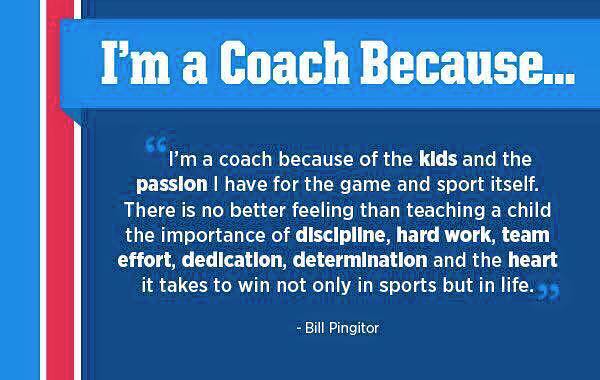The image features a blue background with a vertical stripe on the left side that transitions from bright blue to bright pink. At the top is a horizontal blue ribbon with white font that reads, "I'm a coach because...". Below, in centered white text, is a quote that reads, "I'm a coach because of the kids and the passion I have for the game and sport itself. There is no better feeling than teaching a child the importance of discipline, hard work, team effort, dedication, determination, and the heart it takes to win not only in sports but in life." The quote is attributed to Bill Pingatore, whose name is also centered at the bottom of the text. The important words in the quote such as "kids," "passion," "discipline," "hard work," "team effort," "dedication," "determination," and "heart" are highlighted in bold. The overall design includes a dark blue background beneath the ribbon and on the right side of the image.